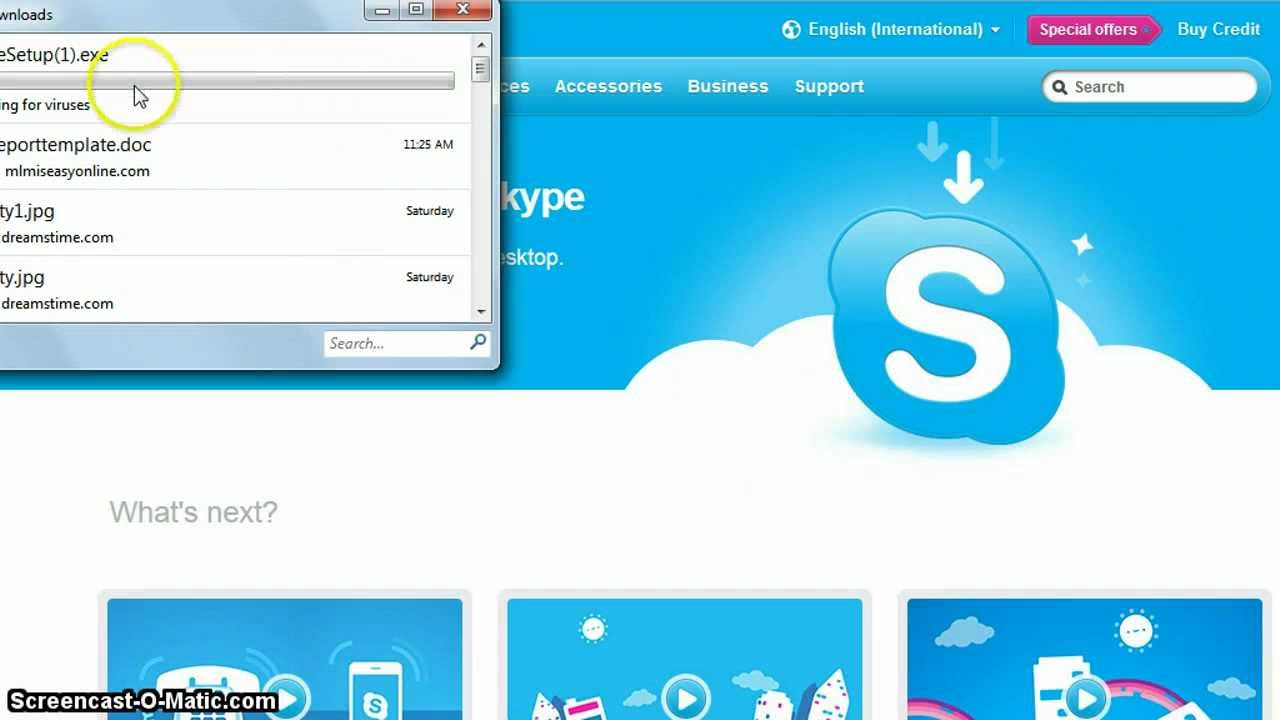This image is a screen capture from a YouTube video tutorial illustrating the process of installing Skype. The tutorial provides a step-by-step guide, beginning with the download of the "SkypeSetup1.exe" file. In the upper right-hand corner of the screen, this specific file is highlighted with a yellow circle around it, and the cursor is pointing to it to draw attention. Despite the initial confusion, the image indeed shows the current downloads rather than a step-by-step process.

The background of the video features a light blue sky with white clouds, incorporating Skype's logo—a white 'S' inside a cloud. At the top of the screen, partially obscured by the download box, are toolbars with options labeled 'Accessory,' 'Business,' and 'Support.' There are also offers such as 'Buy Credit' and 'English International.'

Below the highlight, there are additional tutorial videos indicated by three boxes. Although partially obscured, one of these boxes showcases an old-fashioned telephone icon. The remaining boxes appear to represent video tutorials, each marked with a play button. Overlaid on the screen is the watermark "Screencast-O-Matic.com," slightly obstructing some of the tutorial elements.